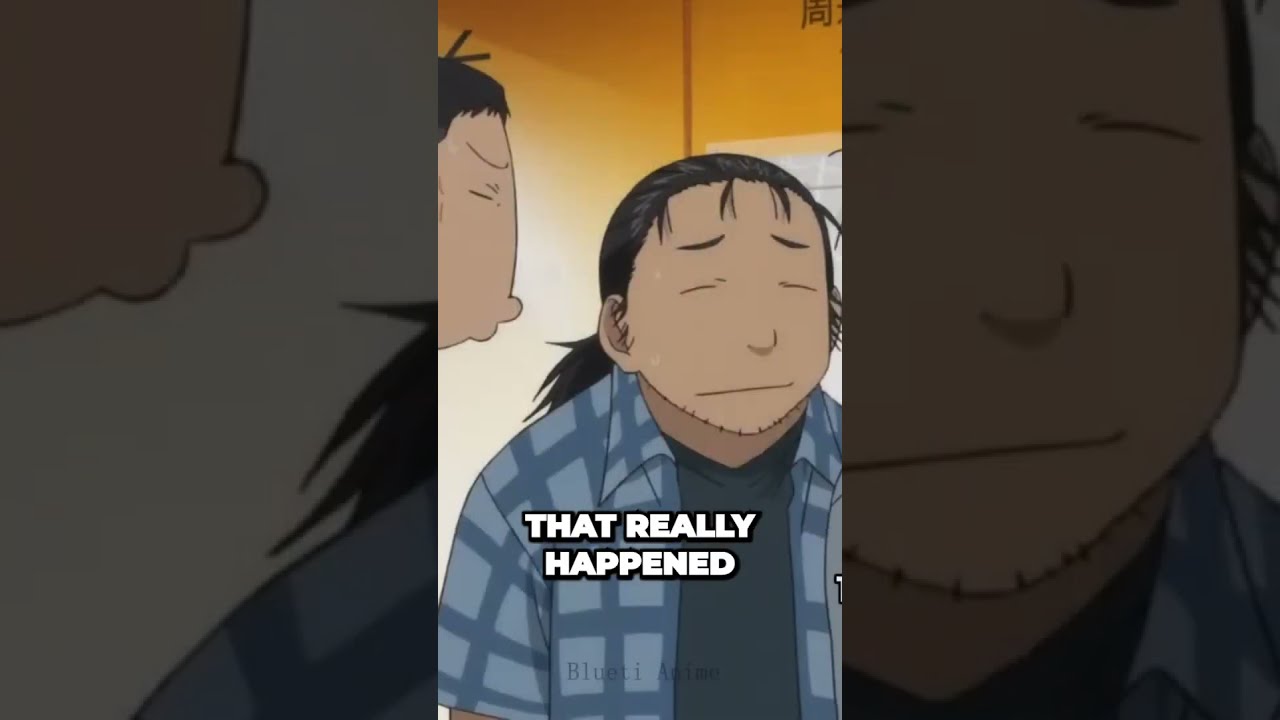In the image, we observe a vertical, cell phone-style snapshot that showcases Japanese anime art. The central frame features an anime-style man with closed eyes, a thin straight mouth, and a light stubble on his chin. His hair is short and cropped, with a small ponytail at the back. He is wearing a blue and gray plaid button-down shirt, unbuttoned to reveal a greenish or dark blue t-shirt underneath. The background consists of an orange wall that transitions to yellow and beige tones, adding dimension to the setting. To the left of the main figure, there is a partial view of another character puckering their lips, with both individuals having closed eyes. Additionally, there are sweat drops on the central man's face, indicating some level of exertion or stress. Overlaying the lower half of the central figure's chest, white text in all capital letters reads "THAT REALLY HAPPENED," providing a contextual clue yet leaving some ambiguity.